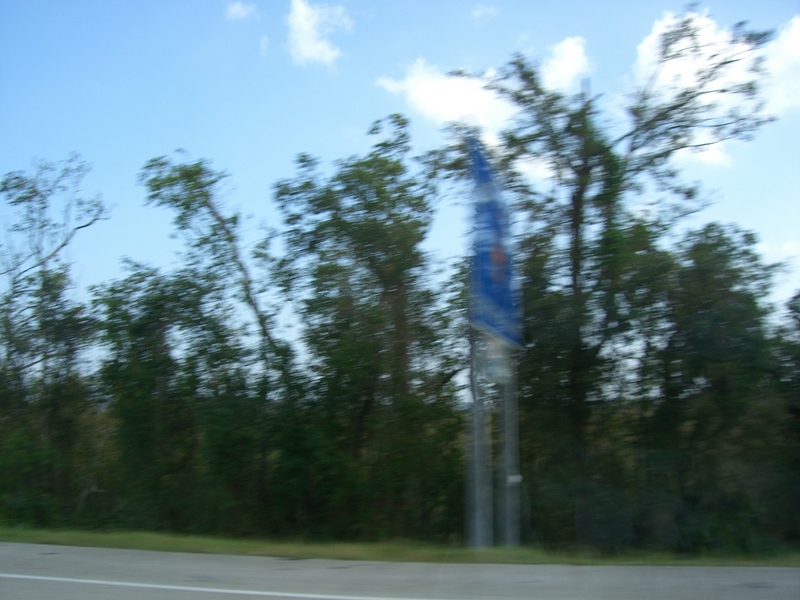This outdoor photograph, taken during the daytime, features a highway scene captured in a landscape format. At the bottom of the image, a portion of the gray pavement of the road extends from left to right, occupying about 10 to 15 percent of the frame. A distinct white stripe marks the edge of the road, denoting the beginning of a light green grassy shoulder where a blue road sign stands. The sign, mounted on two tall metal poles approximately six to ten feet high, is positioned slightly right of center and angled to the right, making its orange middle section and white writing at the bottom barely visible due to the blur and its orientation. The area behind the sign consists of a backdrop of sparse, tall trees with thin branches, set against a bright blue sky dotted with a few white, fluffy clouds, particularly noticeable in the upper right corner. No vehicles are present, leaving the focus solely on the road, the sign, and the surrounding landscape.